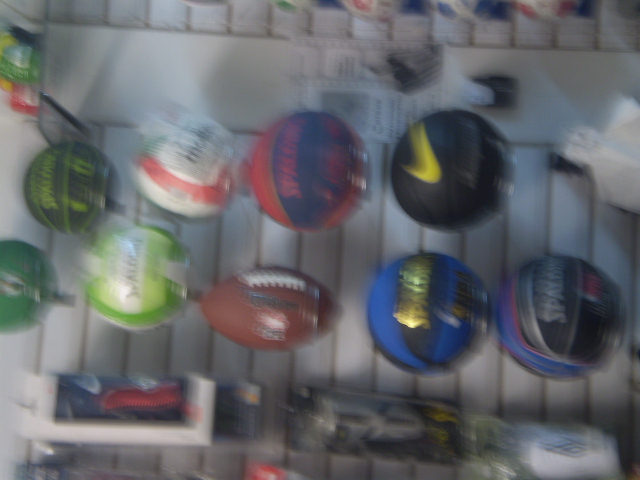The image is very blurry, making it difficult to identify the background, which appears to be a fence or possibly decking. The main focus is on various sports balls arranged in a grid-like formation. In the top left, there are four soccer balls. The top left soccer ball is black and green with the word "Spalding" on it, followed by a green one below, then a white and red one, and another green one beneath that. Next to these soccer balls, there is a blue and red basketball, followed by a football below it. To the right of the football, there is a black basketball featuring a gold Nike swoosh. Further right is a blue and light blue basketball with "Spalding" in gold letters. Rounding out the collection, the last basketball is a combination of red, black, and blue colors. Underneath the balls, there appear to be two packs of items that are indistinct due to the blur. Overall, this image captures an assortment of soccer balls, basketballs, and a football amidst a fuzzy and indeterminate background.